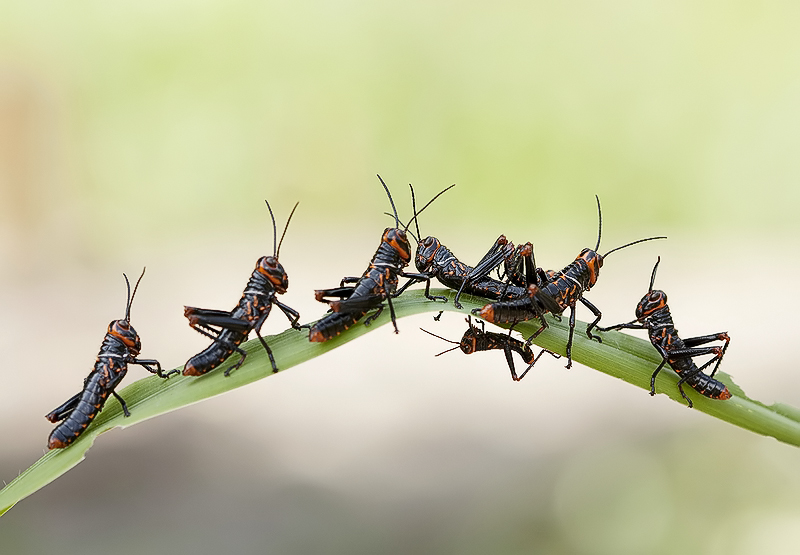This horizontal, rectangular color photograph depicts seven grasshopper-like insects on a large green leaf, which extends across the image from left to right. The leaf inclines slightly upward in the middle and then descends towards the right edge. The background is completely blurred, putting the six large insects and one smaller one in sharp focus. The main insects are primarily black, adorned with vivid orange markings along their heads, lower bodies, and tails. Their upper back legs have black barbs and shiny black feet, with additional orange coloring at their knee joints. The grasshoppers also feature a distinct white ring around their necks. Three of the large grasshoppers on the left side face right, while the three on the right face left, meeting at the highest point of the leaf. A smaller grasshopper clings upside down to the right end of the leaf, and the edges of the leaf show various damaged spots where the insects have been feeding.